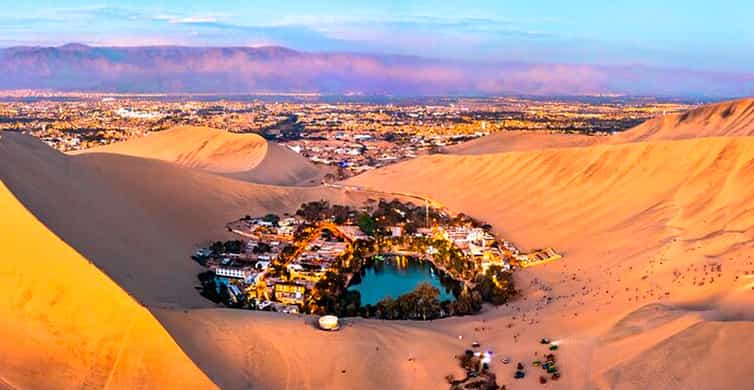This photograph depicts a striking oasis-like city nestled in the middle of a desert landscape. The city, surrounded by sandy hills and dunes, centers around a large pond or lake, which is unusual and striking in such an arid environment. The buildings and structures radiate outwards from this central water feature, creating a concentrated area of greenery amidst the sand. Beyond the immediate cityscape, the surrounding desert continues to stretch into the background, transitioning into larger dunes and eventually a distant mountainous region. The sky overhead is a captivating blend of blue and pink hues, suggesting the image was captured around sunrise or sunset. The scene, whether it is a real photograph or a highly detailed digital illustration, captures the surreal beauty of this unexpected desert oasis against the vast, sprawling sandy terrain.